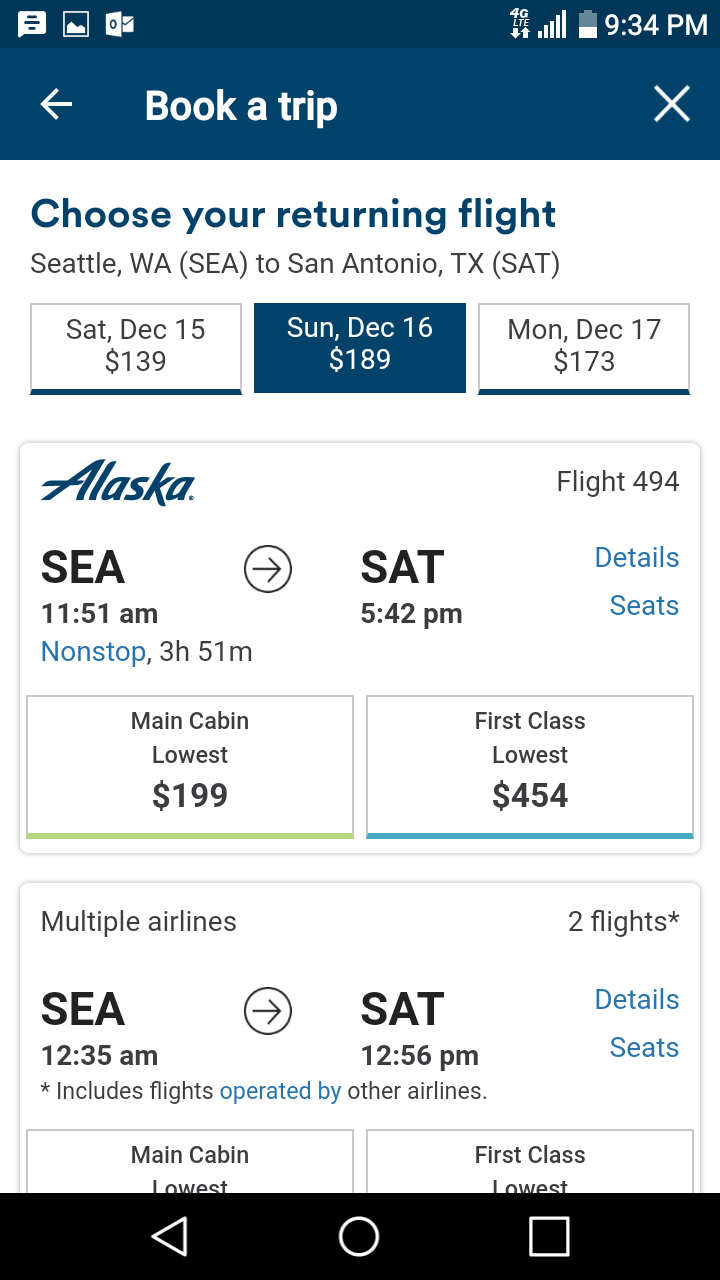The image is a screenshot from an online airline booking service, showcasing options for flights departing from Seattle. The time displayed in the top right corner is 9:34 PM. The booking page offers three flight options: 

- Saturday, December 15th for $139
- Sunday, December 16th for $189 (selected)
- Monday, December 17th for $173

The airline featured is Alaska Airlines, providing a non-stop flight with a duration of 3 hours and 51 minutes. Below the date options, there are two cabin choices available:
 
- Main Cabin for $199
- First Class for $454

The page has a clean, all-white background, emphasizing the flight details and options.